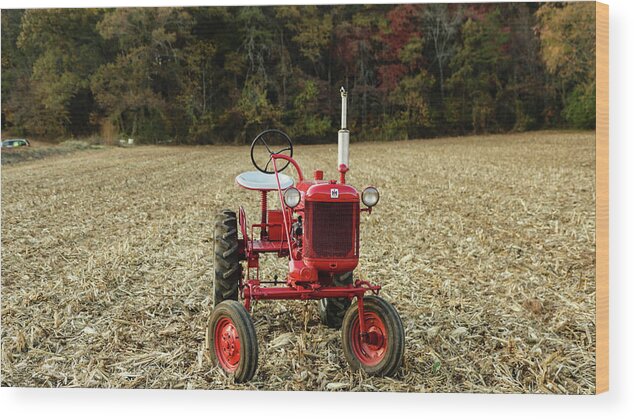This image features an old-fashioned, red tractor situated on a sprawling expanse of dried grass or hay. The vintage tractor, likely around a hundred years old, is open and lacks a roof. It has a distinctive design with smaller black wheels at the front and larger, thin wheels at the back. The vehicle is equipped with a long steering column leading to a black round steering wheel and a white seat. Prominent features include two front headlights, a vertical exhaust pipe, and an engine on the left side with a grill on the front. The background reveals a dense forest with a variety of trees in green, red, and yellow hues. On the left edge of the photo, the tail end of another vehicle is visible, hinting at nearby parking. The photograph appears to be printed on a wooden canvas, adding a rustic charm to the scene captured.